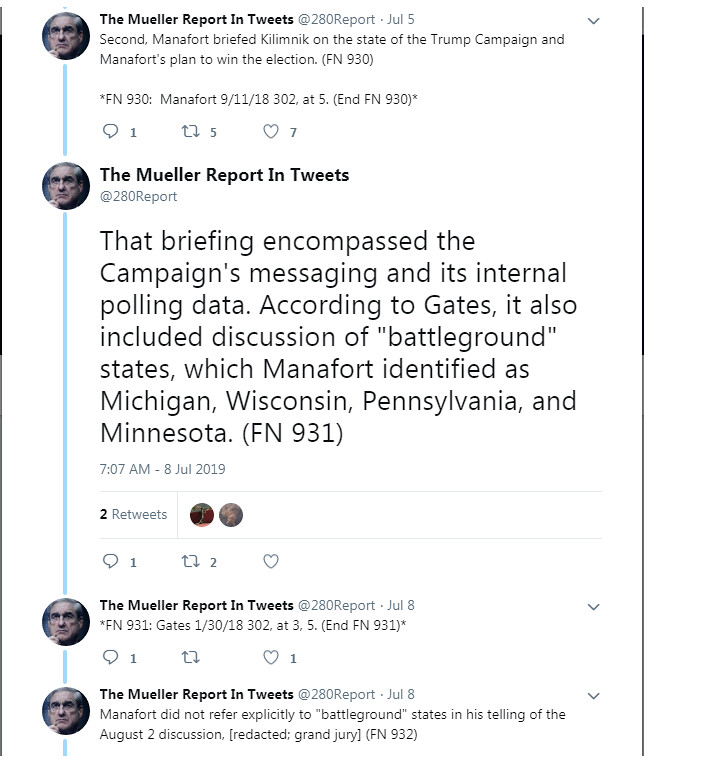The image is a detailed screenshot of several tweets from the Twitter account "Mueller Report in Tweets," with the handle @280report. The account's profile picture features a close-up of Robert Mueller's face. The tweets narrate findings from the Mueller Report, focusing on interactions involving Paul Manafort. The first tweet, dated January 5th, states that Manafort briefed Kilimnik on the state of the Trump campaign and outlined his strategy to win the election, providing intricate details. The subsequent tweet explains that this briefing included the campaign's messaging and internal polling data. Gates, another key figure, noted that the discussion also covered battleground states, specifically Michigan, Wisconsin, Pennsylvania, and Minnesota. The final tweet indicates that Manafort did not explicitly mention battleground states during the August 2nd discussion. Parts of the content are redacted due to a Grand Jury investigation.